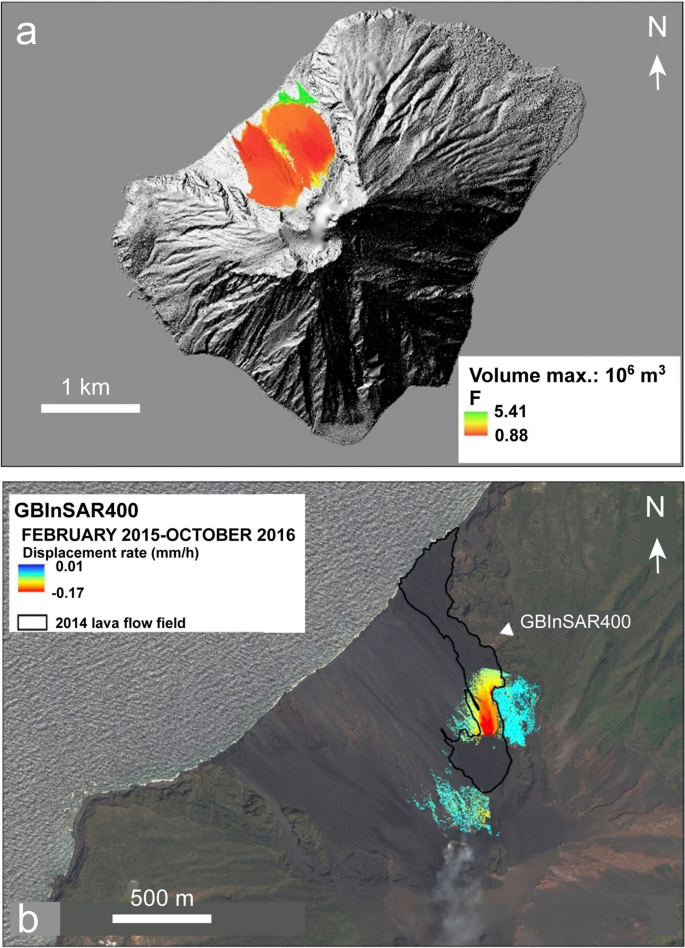This scientific image depicts two stacked 3D terrain models, presumably related to volcanic or geological activity. The top image (labeled 'A') illustrates a textured, black and white rocky terrain, likely representing a volcanic area. It features colored regions in red, yellow, and green, indicating different measurement zones, with a glowing orange cluster on the upper left. The top right includes a north-pointing arrow and a scale legend indicating one kilometer. Additional text includes "volume max 10^6 m^3" and values like "5.41" and "0.88".

The bottom image (labeled 'B') displays a similar rocky terrain with colored overlays—primarily teal, red, and yellow—indicating displacement rates from February 2015 to October 2016. The upper left is labeled "gbin SAR 4000", and the legend specifies displacement values of "0.01" mm to "-0.17" mm. The bottom area outlines a piece of land next to a body of water, showing a 'hot spot' area with the 2014 lava flow field highlighted.